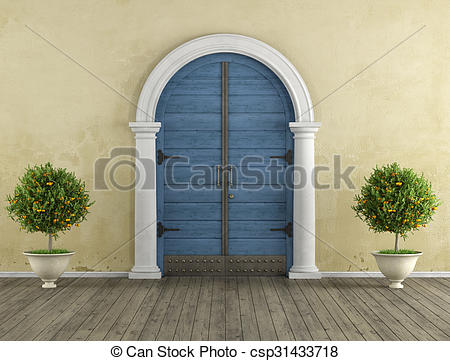The image features an elegant arched entrance with double doors—each door rounded at the top—framed by prominent white columns that support a large arch. The doors themselves are a dark blue, accentuated by dark gray metal trim. On either side of the columns stand decorative plants in pristine white pots. These plants have straight stems leading up to perfectly round, green foliage that appears to bear orange fruits or flowers. The scene is set against a tan wall with a grayish, wooden, deck-style floor beneath. The entire image has a watermark across it, including a drawing of a camera and the words "CANSTOCK" along with the code "CSP314433718," making it clear that this is a stock photo. The setting gives an impression of the front facade of a sophisticated villa or house.